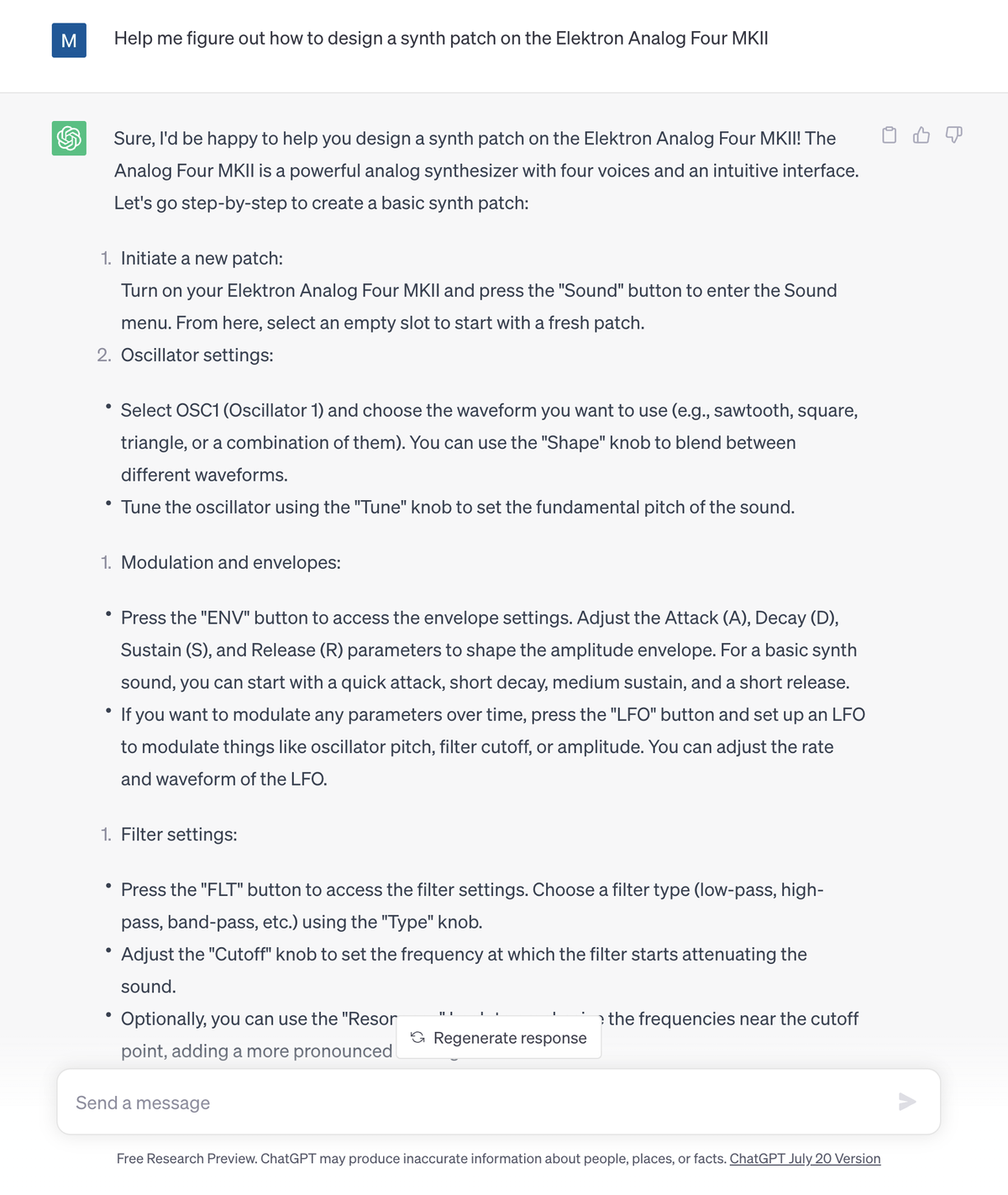The image depicts the ChatGPT interface being used on a device, possibly a tablet or desktop computer, as inferred from the size of the screenshot. The familiar ChatGPT layout is clearly visible, with user questions displayed on a white background and ChatGPT's responses on a gray background.

The user, whose icon is a default blue circle with the letter "M," has asked a question regarding synth patch design on the Elektron Analog Four MK2. This question is shown prominently at the top of the chat interface. ChatGPT's response is comprehensive, spilling over five paragraphs that extend further down in the screenshot, indicating a lengthy and detailed reply. The response follows the standard format, with ChatGPT's green and white logo serving as its icon.

At the upper right corner of ChatGPT's response, typical interactive elements are displayed, including thumbs up and thumbs down buttons for feedback and an additional button for more information on the response. At the bottom of the screen, there's a "Send a message" text input field on a white background, with a send arrow icon that becomes active once the user starts typing.

A floating "Regenerate response" button is positioned towards the lower middle of the chat text, just above the input bar, suggesting the option to generate an alternative response if the current one is unsatisfactory. The overall layout and elements provide a clear and functional user interface typical of the ChatGPT platform.